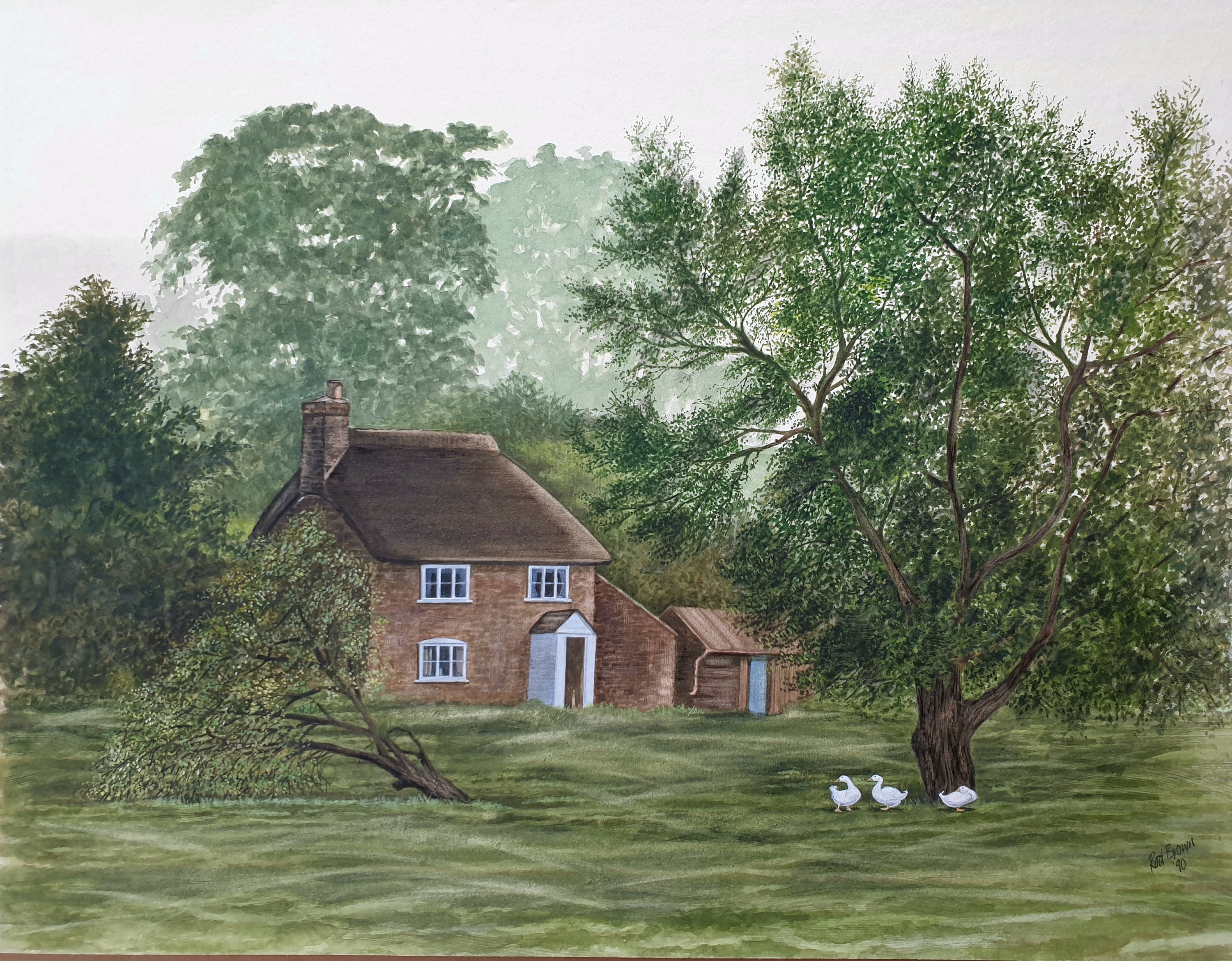This detailed watercolor painting depicts a serene country scene centered around a charming red brick house with a thatch-style roof and a brick chimney on the left side. The house, positioned at an angle, features a white wood entrance with an eaved roof, a small white bay window on the bottom story, and three paned windows on the second floor. Next to the house stands a rustic brown wooden shed with an eaved roof and a blue front door. 

In the foreground, the lush green lawn is home to various trees and wildlife. On the left side, a smaller deciduous tree with a brown trunk and green leaves, adorned with white buds, leans to the left, having fallen on its side. Dominating the right side is a large old tree with a thick brown trunk and numerous Y-shaped branches, creating a canopy of green leaves. Beneath this tree, three white ducks stand on the soft, flowy prairie-like grass, looking towards the fallen tree. 

In the background, several mature trees with dark green foliage rise behind the house, with some showing a mix of dark and light greens and hints of brown. The sky above is depicted in a hazy white, adding to the nostalgic and tranquil atmosphere of the scene. The artist's signature is visible in the lower right-hand corner, completing this picturesque rural composition.